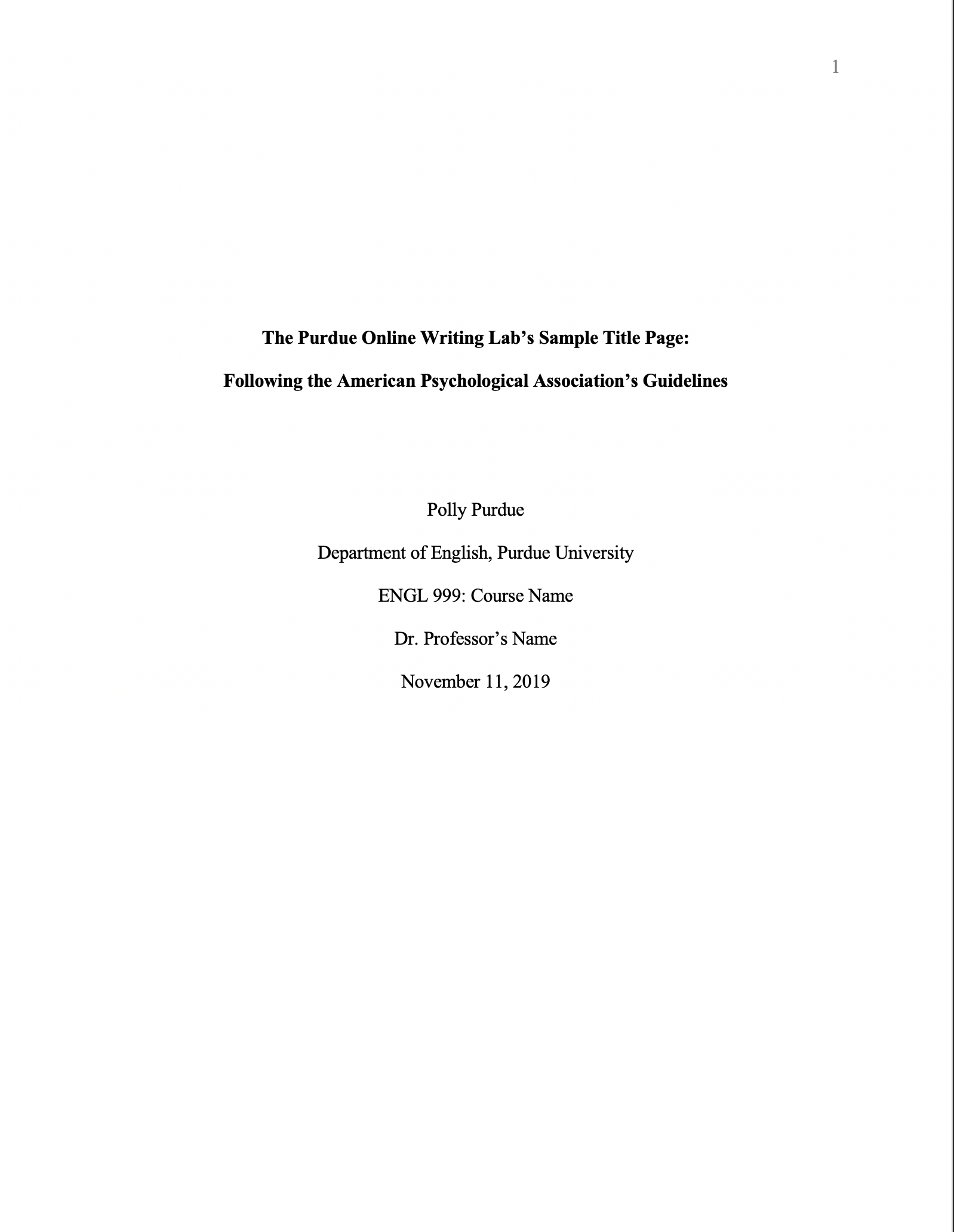The image depicts a sample title page in accordance with the American Psychological Association's guidelines, provided by the Purdue Online Writing Lab. The background is completely white except for a thin black pinstripe running vertically down the right side of the page. In the upper right corner, there is a black numeral "1". The title at the center reads, "The Purdue Online Writing Lab's Sample Title Page: Following the American Psychological Association's Guidelines" in bold black print. Below the title, the following text is centered and in standard black print: "PolyPurdue, Department of English, Purdue University, ENGL 999: Course Name, Dr. Professor's Name, November 11, 2019." The left, top, and bottom sides of the page remain open, giving a clean, minimalist appearance to the document.